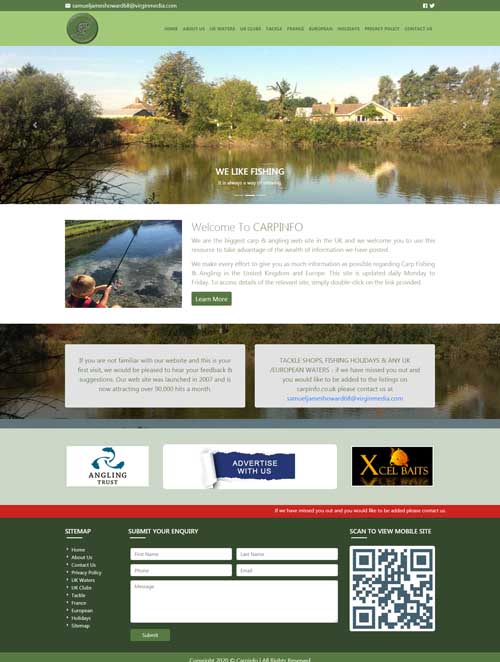The image is a somewhat blurry screenshot of a webpage with a green border at the top. Below the border, there are several clickable areas designed to reveal different pictures and information. The main image underneath these clickable areas showcases a tranquil scene featuring a pond or some other water source surrounded by trees, all set against a backdrop of a blue sky.

In the distance, there is a house with a large chimney on the roof. The text "We like fishing" is displayed prominently, followed by "Welcome to Carp Info". Adjacent to this text, there's a picture of a person fishing.

Beneath this image and text section, there are two paragraphs of descriptive content, accompanied by a green button. Further down, another outdoor scene filled with greenery is displayed. Below this scene, two text boxes appear, each containing additional information.

At the bottom of the image, there are three advertisements, though their specific content is unclear. Below the ads, there is a section where users can enter their personal information to sign up for something. To the right of this signup area, a QR code is visible.